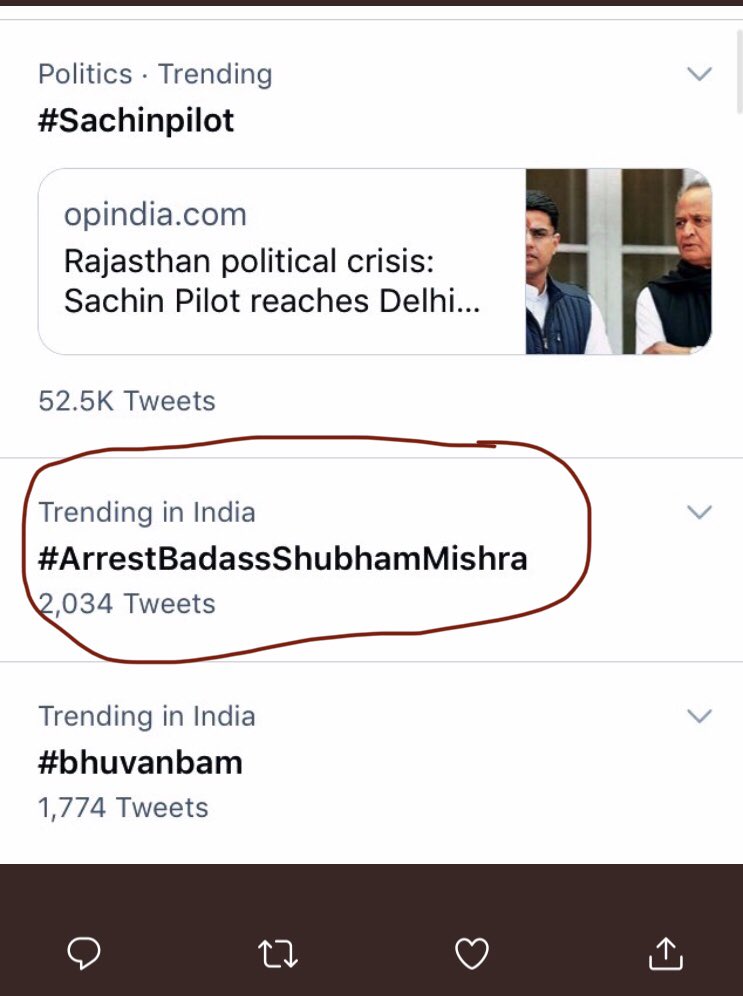This image features a social media post highlighting current political trends and hashtags. It has a predominantly white background with a dark horizontal bar at the top. At the top section, it states "Politics · Trending" in gray text, followed by the hashtag "#SachinPilot" in bold black text. 

Prominently displayed within the image is a rectangular graphic with rounded corners labeled "opindia.com." This portion reports on the "Rajasthan political crisis," noting that "Sachin Pilot reaches Delhi." Beneath this headline, the post indicates there are "52.5K Tweets," along with a note that this trend is happening in India.

Further down, another highlighted section shows the hashtag "#ArrestBadassShubhamMishra" which has generated "2034 Tweets." This part of the post has been circled with a maroon marker, and an arrow pointing downward has been drawn to emphasize it.

Adjacent to this, in a separate trending section, the hashtag "#BhuvanBam" is showcased with "1774 Tweets," also accompanied by a downward-pointing arrow.

At the bottom of the image, a brown box contains a series of icons, including a conversation bubble symbol (suggestive of messaging), an icon with two intersecting lines forming a box, a heart icon, and an upward trending arrow with two ends. These icons likely represent engagement options such as commenting, sharing, liking, and viewing further analytics for the post.

Overall, the image provides a detailed snapshot of trending political topics and hashtags, complete with visual elements to enhance the focus on each trend.